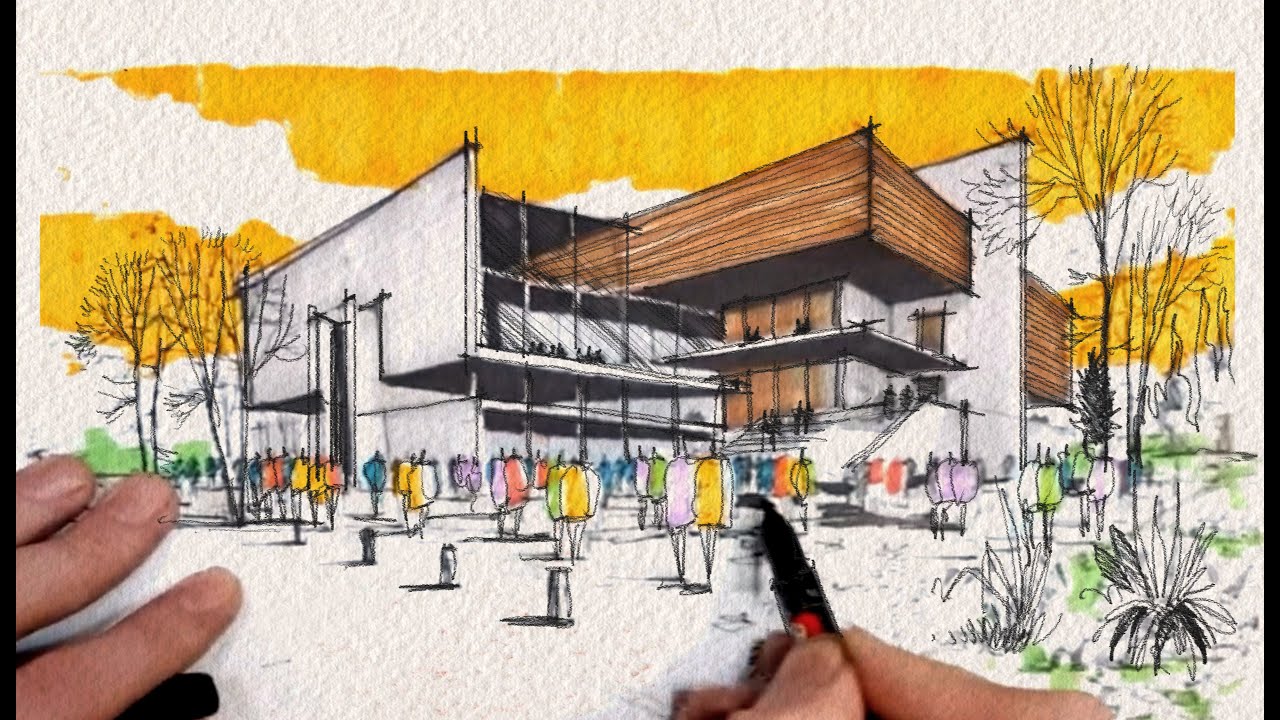This image presents a horizontal rectangular artist's drawing, possibly a proposed architectural project. Framed by black edges, the artwork captures the dynamic process of creation, with the artist's hands visible in the foreground. On the lower left, three fingers hold down the drawing, while on the lower right, the thumb and index finger grasp a black pen—actively sketching details. The depicted building is strikingly modern, characterized by white walls, expansive windows, and wood balconies. At its entrance, a prominent doorway stands surrounded by leafless trees, indicating a winter scene. The building, reminiscent of a university campus, is three stories tall with a glass front, and numerous colorful figures—dressed in vibrant yellows, purples, and pinks—are shown walking toward it. The sky above is a blend of yellow and white hues, and a hint of greenery is visible in the background.